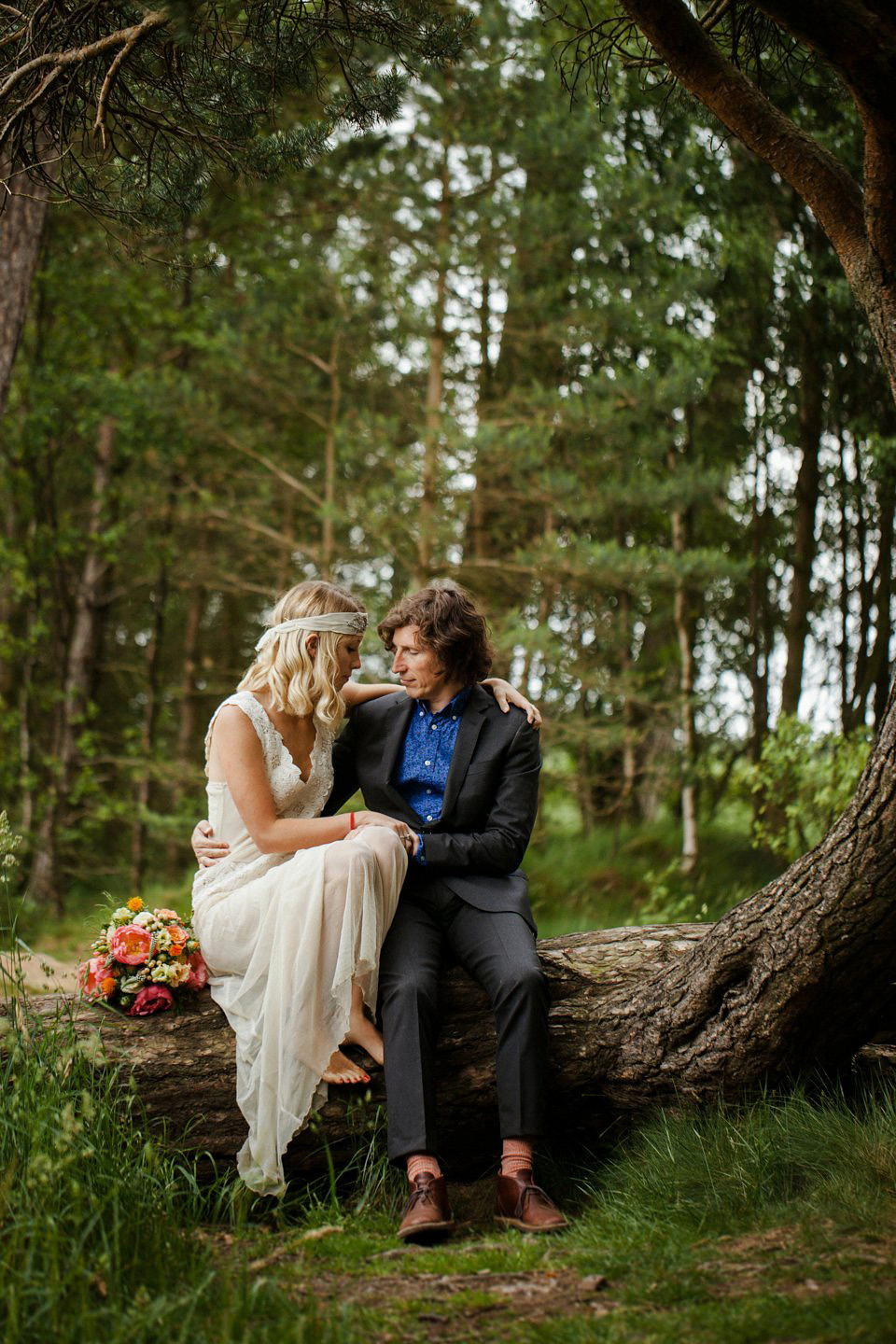In a serene forest setting, a bride and groom are captured in a color photograph, seated on a large, fallen tree trunk. Surrounding them is a lush backdrop of grass and tall trees. The bride, with her long, wavy blonde hair adorned with a white bandana, is dressed in an elegant white v-neck lace dress. Her bare feet rest comfortably on the trunk, and her simple yet ethereal look is accentuated by a red string bracelet around her wrist. Beside her, a vibrant bouquet of pink, white, and orange flowers rests on the trunk. The groom sits closely, his medium-length brown hair adding to his relaxed demeanor. He wears a dark suit with brown shoes and distinctive pinkish-peach socks, paired with a blue button-down shirt, opting for a casual, tie-less look. The two share a gentle embrace, with the groom gazing affectionately at the bride, conveying an intimate and whimsical moment in nature.